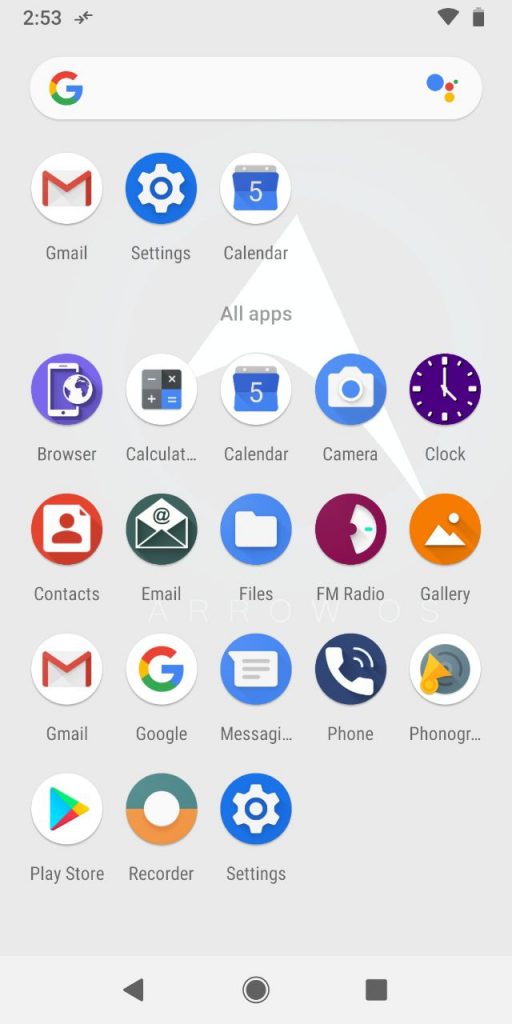Screenshot of a smartphone's app menu taken at 2:53 PM. The screenshot shows a Wi-Fi connection, almost full battery, and an active file transfer. A Google search bar is positioned at the top of the screen. Below it, app icons are displayed in a grid, listed from top to bottom and left to right: Gmail, Settings, Calendar, All Apps, Browser, Calculator, Calendar, Camera, Clock, Contacts, Email, Files, FM Radio, Gallery, Gmail, Google, Messaging, Phone, Phonograph, Play Store, Recorder, and Settings. At the bottom of the screen are the standard Back, Home, and Menu navigation buttons. The image captures the complete All Apps page on the phone.